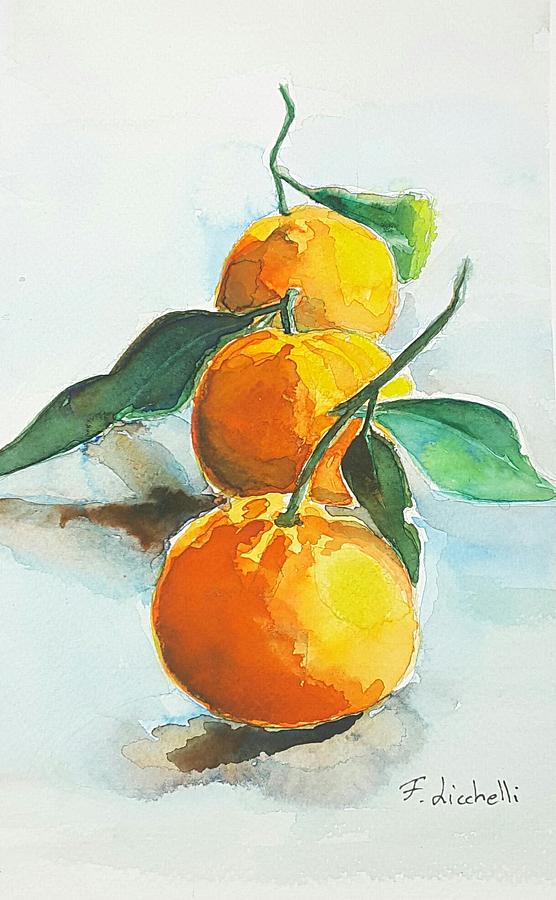This professionally done watercolor painting portrays three pieces of citrus fruit, likely oranges, arranged in a vertical line receding away from the viewer. Each fruit is rooted upright on a non-discriminative, homogenous gray surface with visible shadows cast to the left in dark brown and black watercolor. The table they rest on blends seamlessly with the light greenish-blue background. The frontal citrus fruit has the longest green stem with two leaves attached, painted in light green and dark blue hues. The middle fruit, with a shorter stem and one large leaf protruding to the left, displays a dark orange color with yellow and lighter orange highlights, particularly on its right side. The farthest fruit has a medium-length stem with a single leaf off to the right. A subtle splattering of watercolor in lighter orange and blue extends around the fruits, hinting at a broader shadow. The painting, adorned with a handwritten signature by F. Lucelli in the bottom right corner, is encased in a notably long, vertically oriented frame, adding to its artistic sophistication.